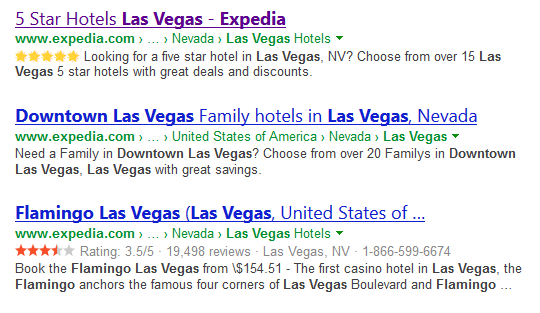The image is a screenshot of search results on Expedia for hotels in Las Vegas. The first result is highlighted in purple, indicating it has been clicked on before, and features "Five Star Hotels, Las Vegas" from Expedia. The link displayed is "Expedia.com," and the description encourages users to choose from over 15 five-star hotels in Las Vegas, Nevada, offering great deals and discounts. 

The second listing is for "Downtown Las Vegas Hotels" and "Las Vegas Family Hotels" in Las Vegas, Nevada. The link, also from "Expedia.com," and the associated text describe savings for families visiting Downtown Las Vegas, with over 20 options available.

The third entry is for "Flamingo Las Vegas," rated at three and a half stars, again from Expedia. This result is also located in Las Vegas, Nevada, and appears under "Las Vegas Hotels."